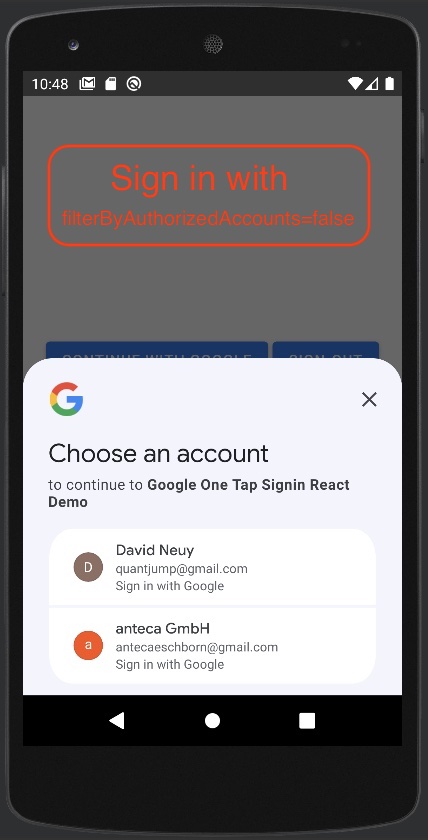This screenshot, taken from a phone, features a login screen with clear visual elements. At the top of the screen, a red rectangle contains the warning message "Sign in with filter by authorized accounts equals false" prominently displayed against a gray background. Surrounding the entire gray background is a border formed by a red rectangle with smoothly curved edges.

Beneath this, a white section signifies the login prompt, beginning with a capital "G" representing Google Chrome at the uppermost part, accompanied by a gray "X" icon for closing the prompt. The text "Choose an account to continue to Google One Tap Sign-In React Demo" follows.

In this section, there are two user account options. The first account is labeled "David Newey," indicated by a "D" inside a brown circle. The second account is "Antica GMBH," marked by an "A" in an orange circle.

At the very bottom of the screen, a black bar holds three navigational icons: on the left is a white triangle pointing to the left, signifying a back button; in the center is a white circle, likely indicating the home button; and on the right, a white square probably representing the app switcher.